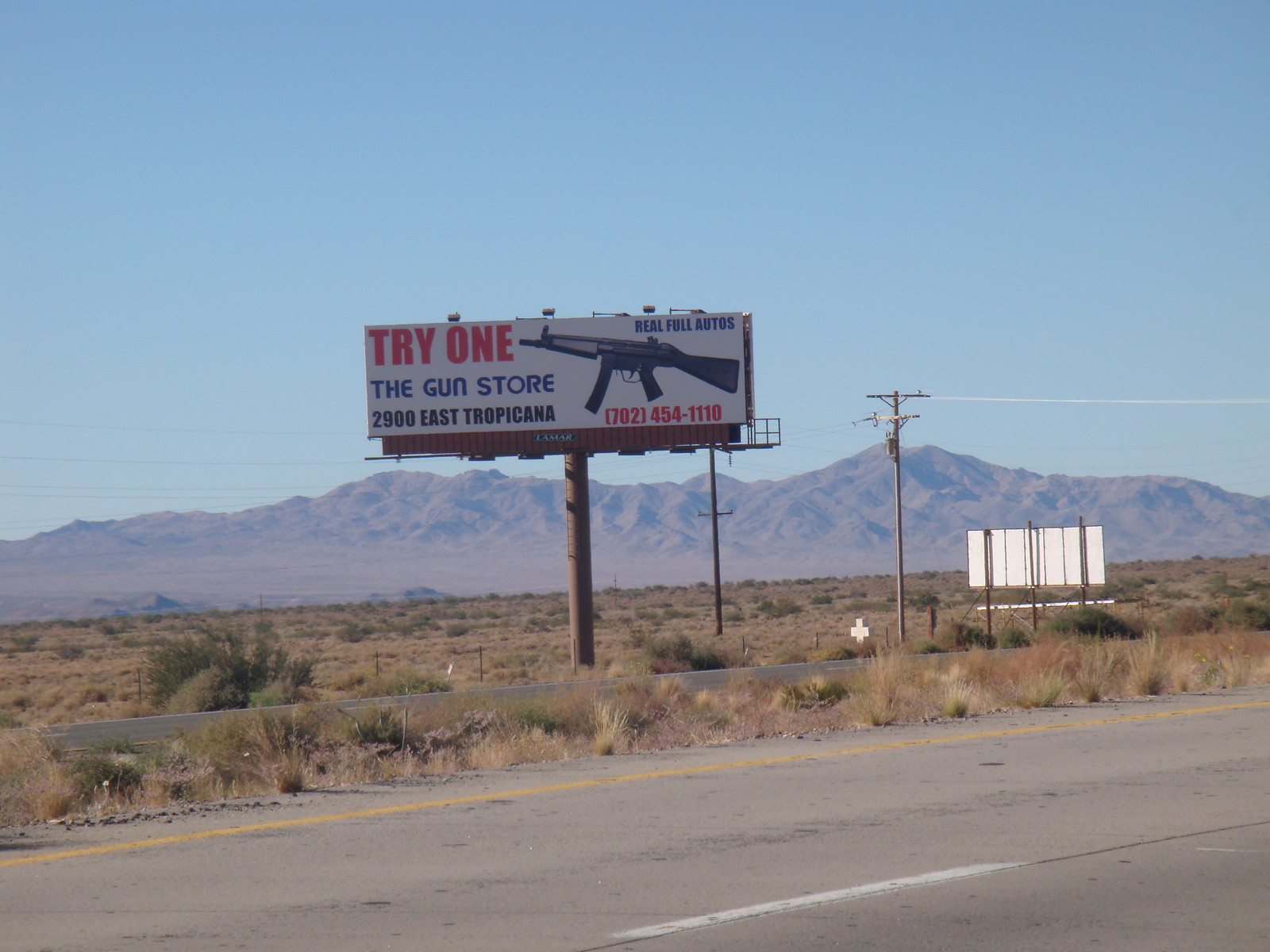The image depicts a desert highway lined with dry, brownish-gray pavement featuring a white line in the middle and a yellow line along the edge. Short, sparse vegetation and dirt occupy the foreground, transitioning into a brownish landscape. Two billboards are visible: one shows its plain white back, while the other faces the viewer. The latter, mounted on a wooden post, advertises in bold letters: "Try One" in red, "The Gun Store" in blue, "2900 East Tropicana" in black, and "Real Full Autos" at the top in blue. An image of a black assault rifle adorns the sign, with a phone number "702-454-1110" in red underneath. Telephone poles and wires also dot the scene, and distant, purplish hills rise against a clear blue sky, completing the desolate yet striking landscape.